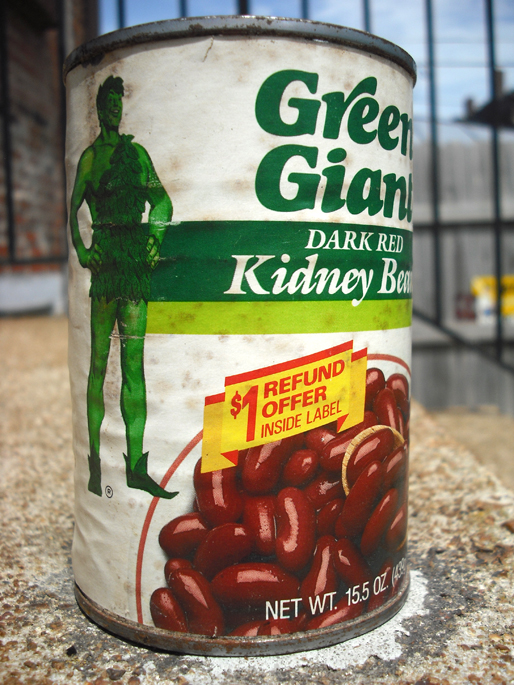The image showcases a can of Green Giant Dark Red Kidney Beans. Featured prominently on the label is a muscular man wearing a leopard-print tunic, striking a confident pose with his hands on his hips and his arms angled outward at approximately 45 degrees. He has curly hair and is smiling warmly at the camera. To the right of the figure, a horizontal green banner stretches across the can, underneath which another banner advertises a "One Dollar Refund Offer Inside Label." Below this text, a bowl brimming with dark red kidney beans is displayed, adding a vibrant touch of color to the label.